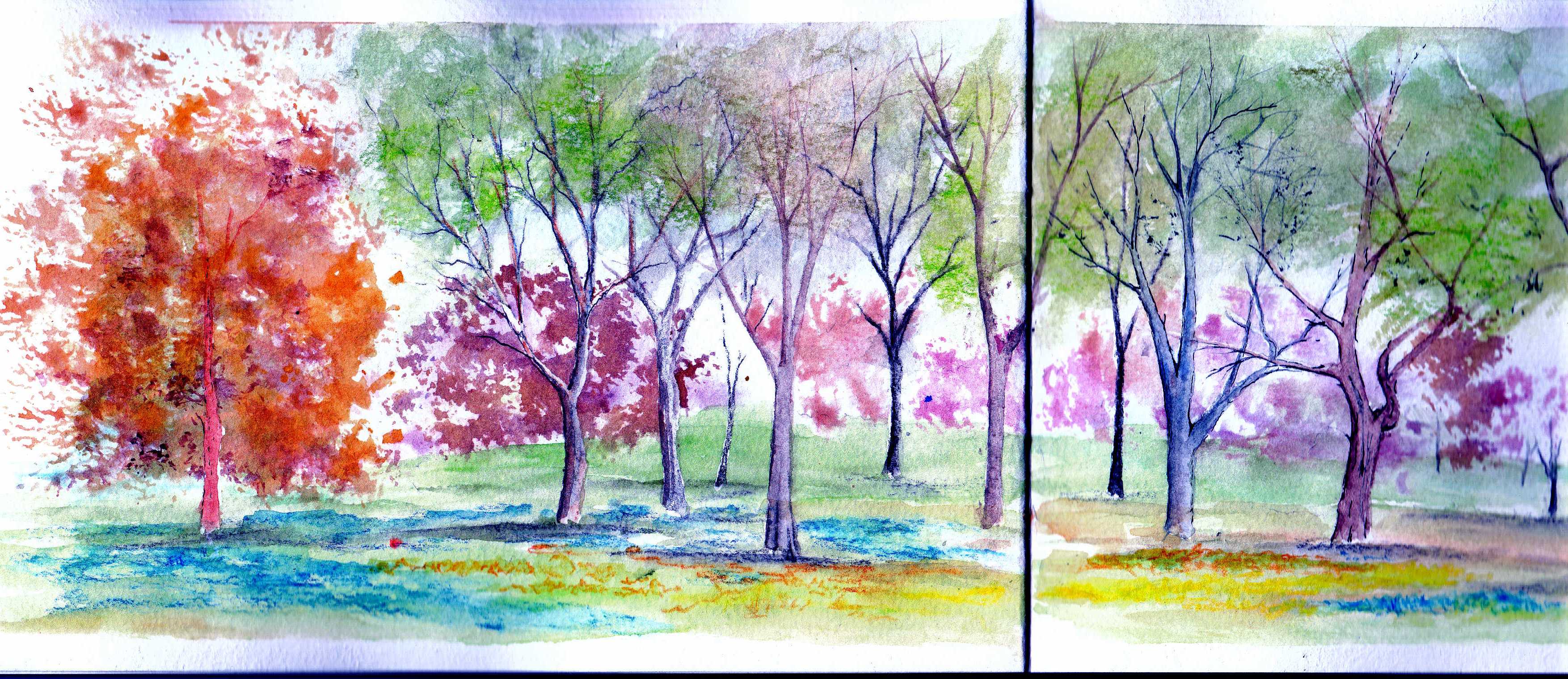This is a detailed watercolor painting that spans across two connected pages, evident by a black line about three-quarters of the way from the left. The scene depicts a variety of trees set against a complex and colorful landscape. On the far left stands a striking tree with bright orange leaves and pinkish branches. The grassy ground below is a mosaic of green, blue, and yellow, speckled with brown. As the painting moves right, several other tall, thin trees come into view with brown or purple trunks. They display varying leaf colors including green, brown, and purple, concentrically clustered towards the top. A noticeable purple border cuts halfway through the painting vertically and extends horizontally along the bottom. The distant background is filled with additional trees and bushes in shades of purple and pink, adding depth and a dreamlike quality to the overall scene.